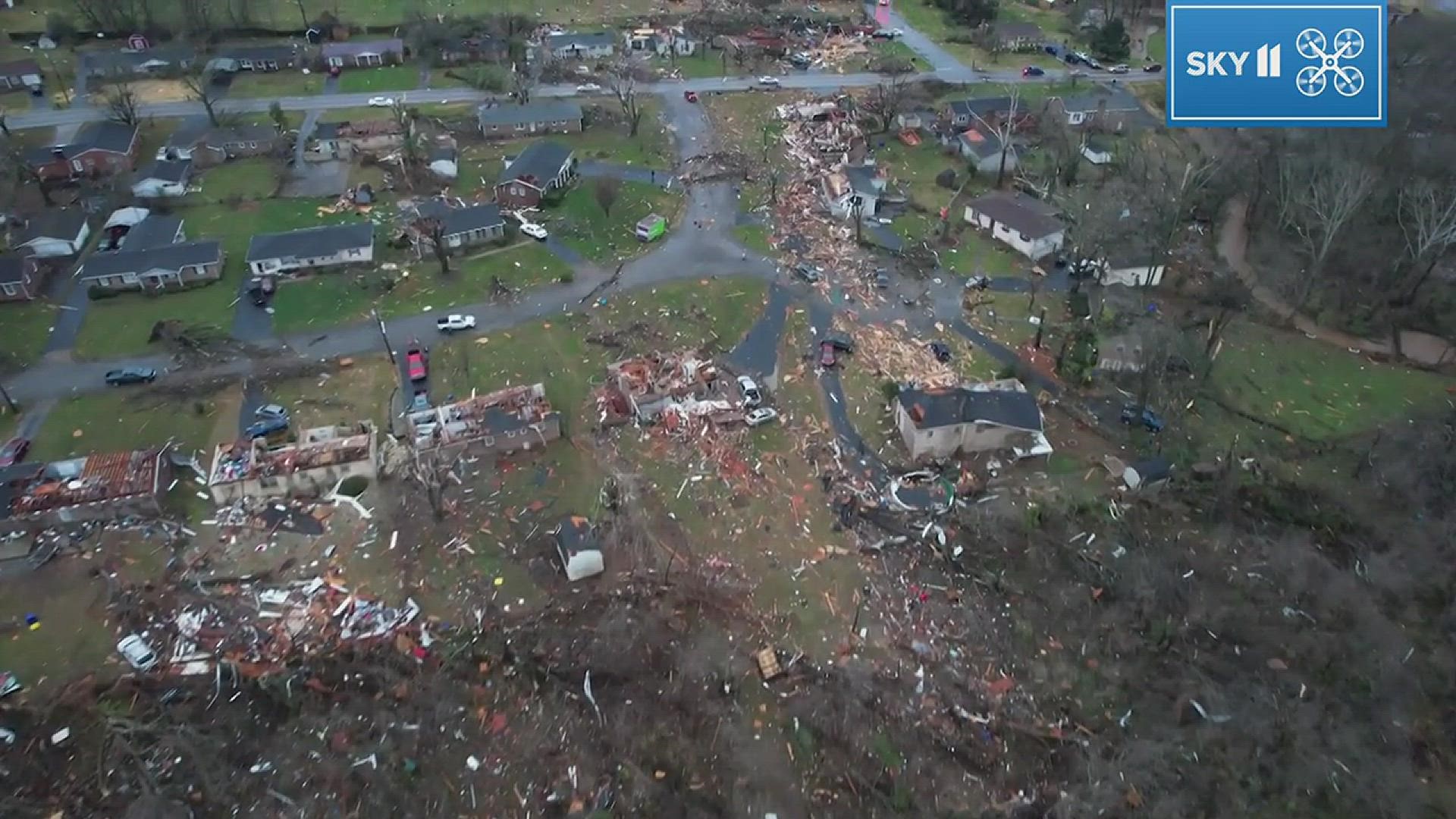This aerial photograph, likely taken from a news helicopter and labeled "Sky 11" in the top right corner, captures the devastating aftermath of a tornado cutting through a typical American suburban neighborhood. From the bottom left to the top center of the image, a clear path of destruction is visible, characterized by splintered homes and scattered debris including wooden planks, cars, and household belongings. Many houses along this path are entirely demolished, their roofs ripped away, while others sustain varying degrees of damage. In contrast, homes toward the top left of the frame appear mostly intact, with some showing minor roof damage. The scene is set against an overcast, gray sky, and dotted with leafless brown trees, suggesting the season is either spring or fall. Driveways with parked cars and a curved road are also visible in this detailed and tragic depiction of a tornado's destructive power.